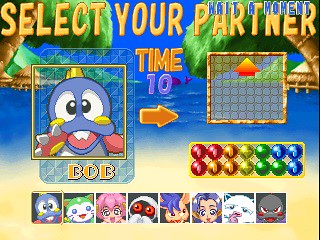This screenshot, captured from a video or arcade game, displays an engaging scene set against a beach backdrop. At the bottom, golden sand transitions seamlessly into the serene blue waters at the center, while a few lush trees in the background add a touch of nature's diversity. Dominating the top of the screen is the message "Select your partner" in eye-catching yellow lettering, indicative of a character selection phase. Just above this, in the very upper right-hand corner, the words "Wait a moment" in blue suggest that the game is currently in a pause state, likely awaiting action from Player 2.

Centrally positioned on the screen, the desperate countdown is underscored by the word "Time" in bold orange letters, with the number 10 in blue displayed beneath it. An orange arrow below these time indicators adds a sense of urgency to the scene. On the left-hand side, the selected character, named Bob—possibly a blue dinosaur—stands prominently. Below Bob, a grid comprising eight smaller squares shows alternate character options available for selection.

To the right of the image, five differently colored gems—red, orange, yellow, green, and blue—are aligned vertically, with an empty square perched just above them, perhaps indicating a slot for collecting or combining these gems. The overall composition and the elements on the screen suggest an immersive and colorful gaming experience, rich with choices and strategic elements.